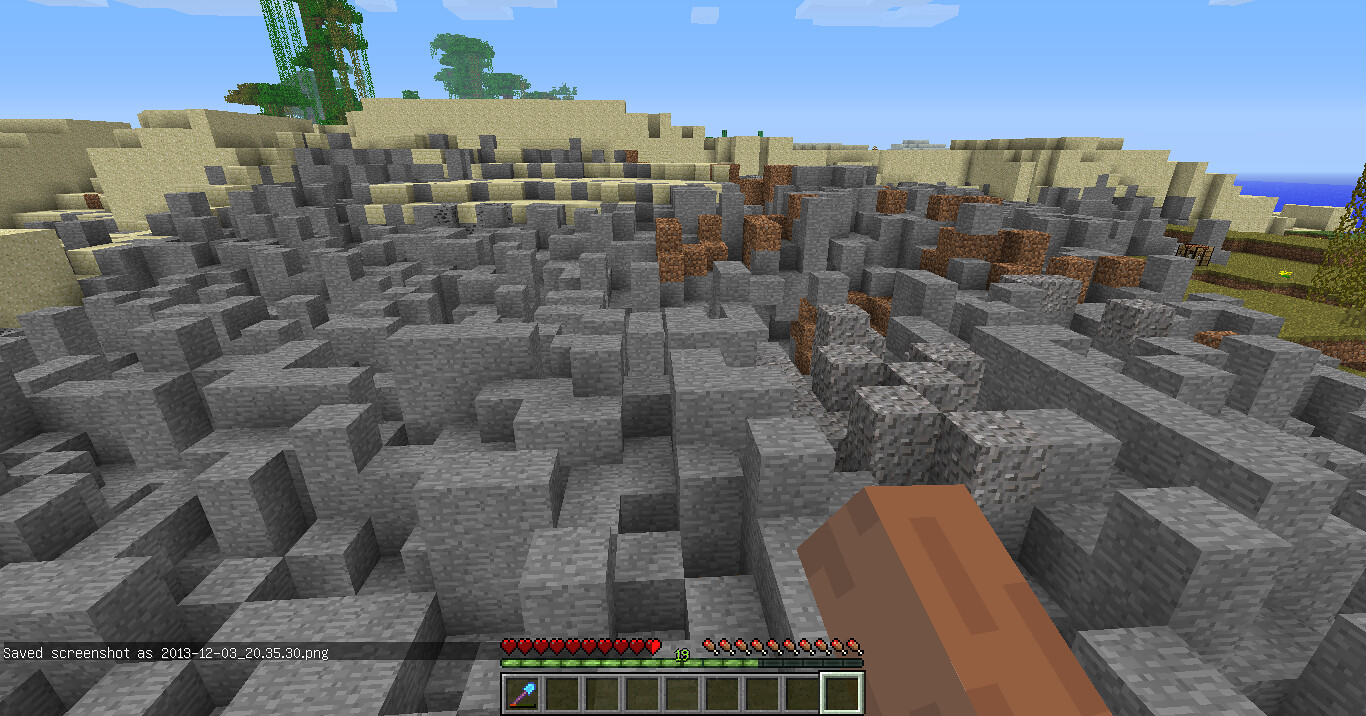This is an image from an old-style video game, likely a screenshot from Minecraft, dated December 3rd, 2013. The HUD at the bottom displays a score block and a row of red hearts. The main scene depicts a cityscape crafted from variously sized stone blocks, stacked at different levels to create a maze-like structure. These cement-colored blocks in the foreground transition into sand-colored blocks towards the back. Higher still, there's a scattering of blonde wood-colored blocks. To the right, the landscape reveals an ocean and some distant trees, under a vivid blue sky with white clouds. The layout suggests a game environment where characters might navigate or jump across the heights and gaps between blocks.